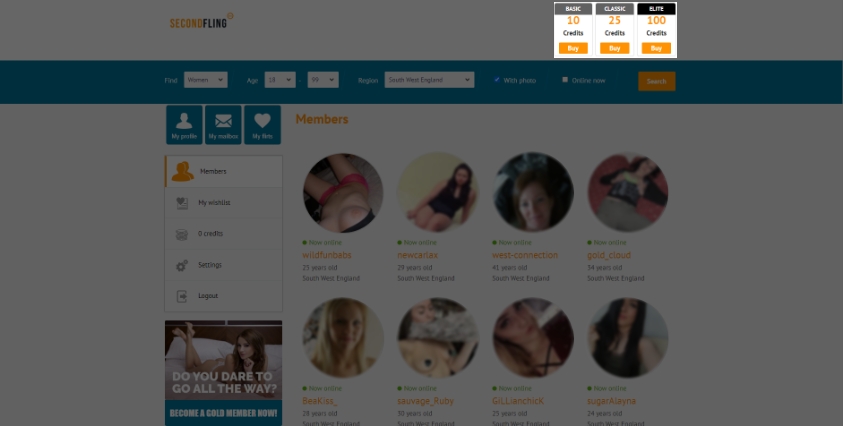The image depicts a dark-themed web page interface titled "Second Fling." At the top section of the page, navigational links are displayed, including options such as "My Profile," "My Matches," and "My Turn." Along the side, there are labeled sections for "Members," "My Wish List," "Credits" with an indication of zero credits, "Settings," and "Log Out." 

The main content area features a grid of user profile pictures, arranged with four images in the top row and four in the bottom row. Overlaying the dark background is a bright white pop-up window divided into three segments, each representing different credit purchase options. The leftmost segment shows "Basic Credits" priced at 10 credits, the center segment displays "Classic Credits" priced at 25 credits, and the rightmost segment lists "Elite Credits" priced at 100 credits. Each segment includes an orange "Buy" button in the bottom corner.